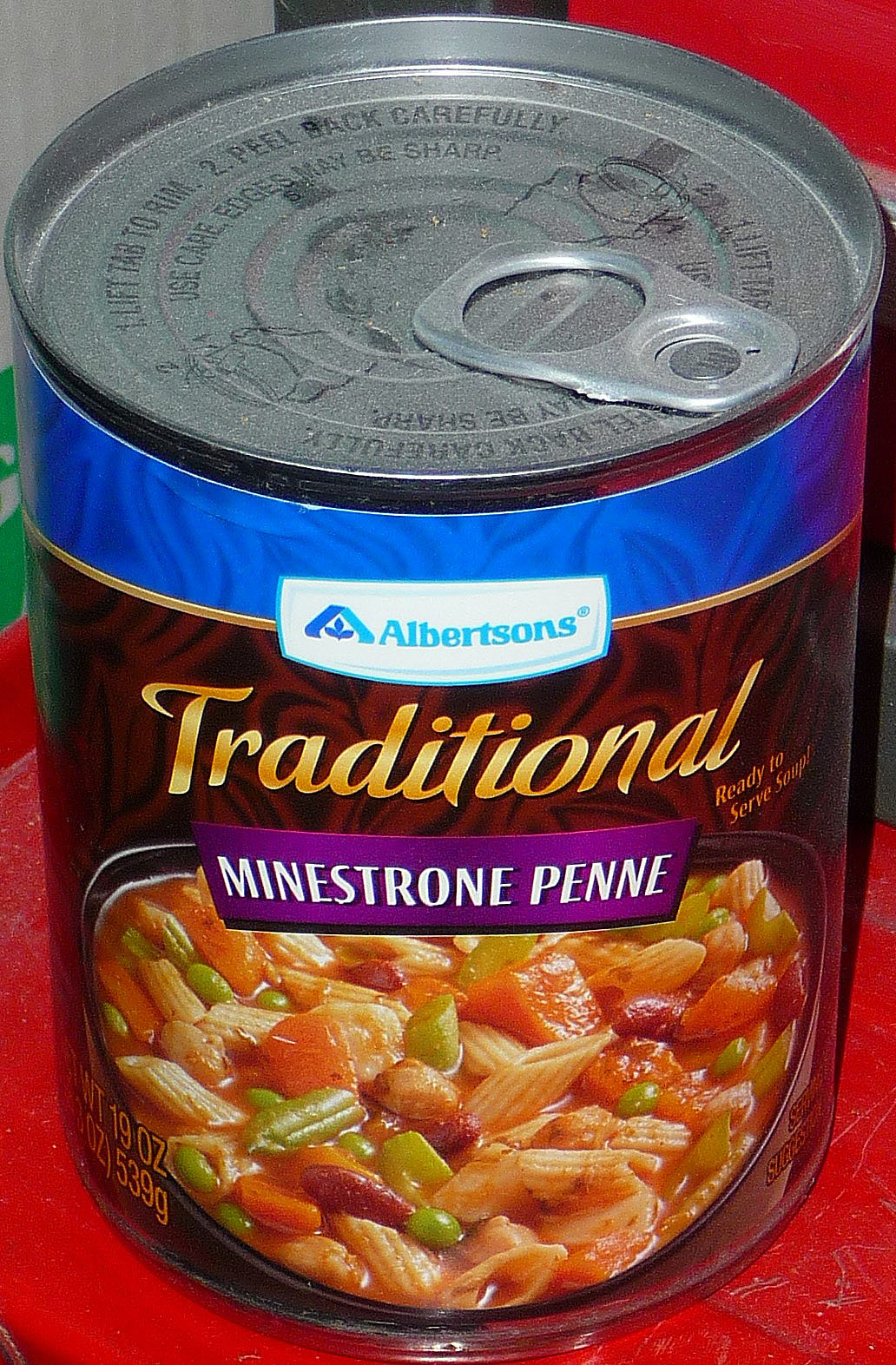Here's a cleaned-up, detailed caption based on the provided voice description:

---

This image features a can of Albertson's Traditional Minestrone Penne Soup. The label prominently displays the text "Traditional Minestrone Penne," with "Traditional" written in elegant gold script and "Minestrone Penne" set against a purple banner. The Albertson's logo is housed in a box at the top of the label, situated below a royal blue band encircling the can's upper edge. The background of the label is primarily brown, adorned with subtle swirling patterns.

Additional label details include "Ready to Serve Soup" text and a notation of the net weight: 19 ounces (539 grams), located in the bottom right corner. The can is equipped with a pull-top lid and appears to be somewhat dusty and dated, indicating it may not be a recently produced item.

The can is placed on a red table, which also has a layer of dust. In a close-up view of the soup within the image, the contents are displayed in a rustic brown crockery bowl, showcasing the minestrone's hearty ingredients—penne noodles, green beans, kidney beans, tomatoes, and celery.

---